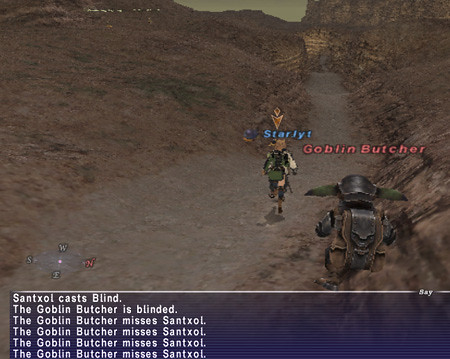This screenshot captures a moment from a video game. At the bottom of the screen, a series of blue notes outline an exchange: "Sense Exhale" is cast, and the Goblin Butcher is blinded. Subsequently, the Goblin Butcher attempts to strike a character named Sam Straw but misses each time, repeating this sequence four times without success. 

Visually, the Goblin Butcher resembles Obi-Wan Kenobi, adorned in military leather armor and carrying a backpack, standing on a rocky ridge overlooking a winding path. The landscape is predominantly arid and desolate, characterized by various shades of brown. The sky, the path, and even the characters blend into this earthy palette, contributing to the barren atmosphere. The path, visible snaking below the rocks, showcases the inhospitable, desert-like environment devoid of any signs of life. The contrasting brown tones of the terrain emphasize the isolation and bleakness of the setting.